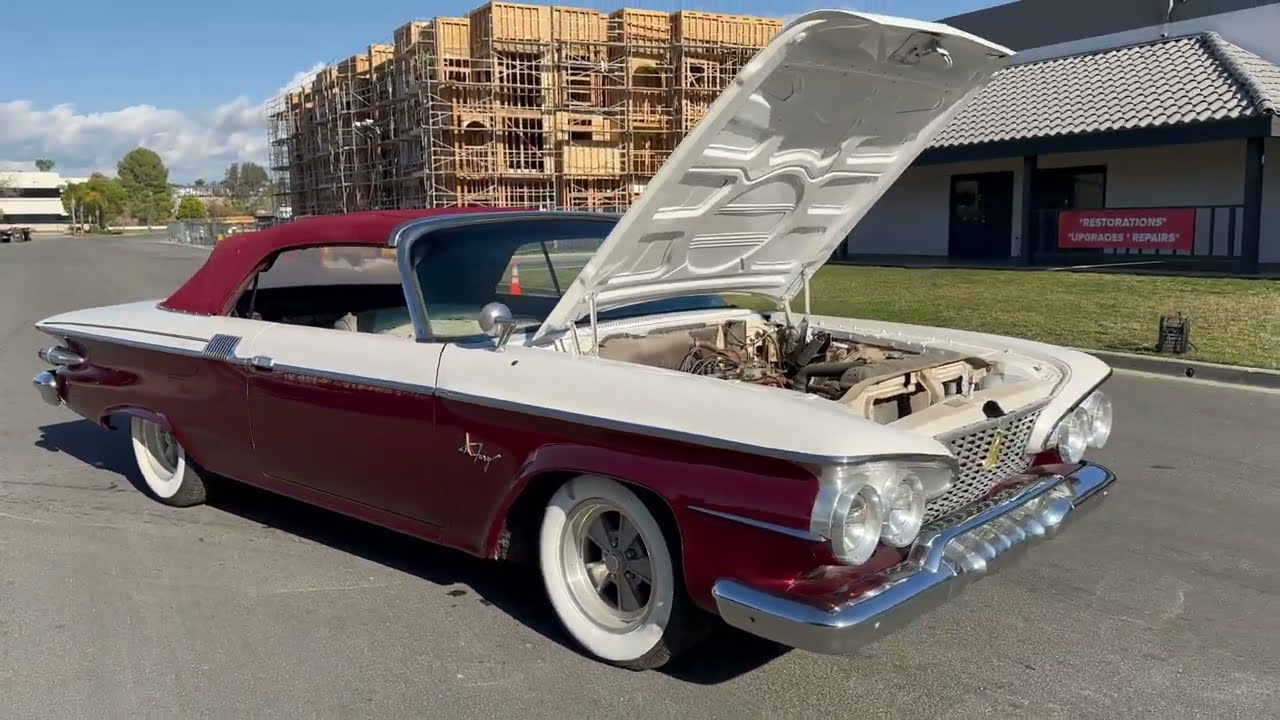This photo captures a classic maroon convertible parked diagonally on an asphalt street during the day. The car, with its hood popped open revealing the engine, features cream-colored accents along the sides and a matching maroon cloth top that is currently up. The vehicle also boasts white wall tires and an indistinct logo or writing near the front right tire. The scene is set outdoors, with several buildings in the backdrop. Dominating the background is a multi-story building under construction, in shades of beige and brown. Further back, various office buildings and trees are also visible. A red sign attached to a black fence in the distance advertises restorations, upgrades, and repairs. The setting blends the classic aesthetic of the car with the bustling environment of urban development.